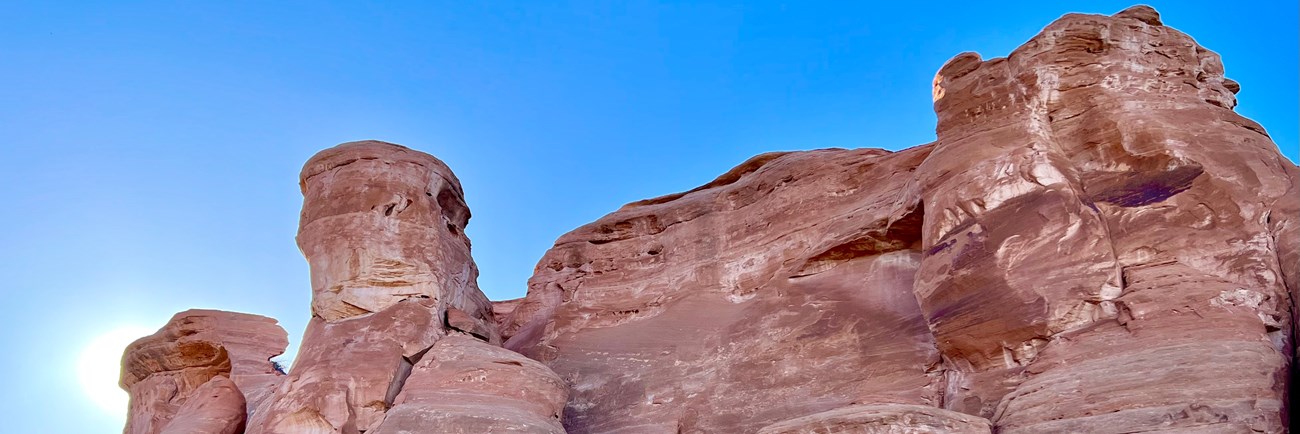The photograph captures a stunning scene of reddish-rock cliffs, likely from a national park or desert region such as Arizona. The rock formation dominates about two-thirds of the frame, with a distinctive light orange hue interspersed with white and darker red layers that reveal the geological lines formed over time. On the left side of the image, two prominent rock projections rise, resembling chimneys, partially obscuring the bright white glow of the Sun as it peaks out from behind the rocks. The sky above is a gradation from the deep blue at the top to lighter blue near the Sun. To the right of the image, a broad, smoother section of the cliff is marked by a brown blotch, possibly a stain from water. Above this is a series of slits and openings, hinting at small caves. The overall texture of the cliffs appears mostly smooth, with noticeable bulges and layers, indicating the erosive processes that shaped them. The photograph perfectly captures the serene beauty of the rugged terrain under a bright, clear sky.